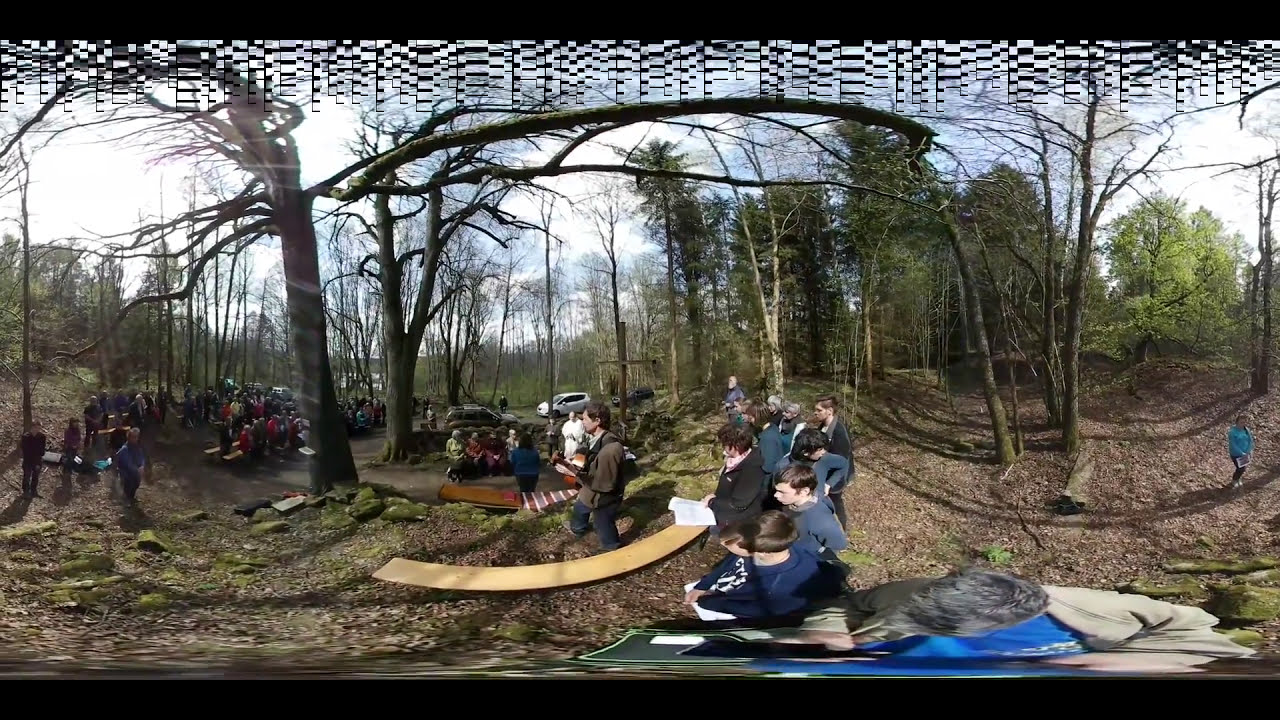The image depicts a vibrant outdoor gathering, likely at a campground set in a forested area. The scene is framed through a fisheye lens, contributing a unique, distorted effect with strange patterns reminiscent of fish gills at the top and a blurred bottom edge. The forest consists of large deciduous trees, mostly bare or sparsely covered with dead leaves, indicating a winter or early spring timeframe. Mixed among them are a few green deciduous trees or evergreens, suggesting a variety of tree types.

In the foreground, there are clusters of children and male adults dressed in sweaters and warm clothing, hinting at the chilly weather. A dozen or so individuals are oriented right to left, appearing to watch an event or focal point out of view. Some people are gathered closely together, and one can be seen holding a sizable open book.

To the left of the image, more people are congregating, with some seated on benches. A couple of vehicles, including a white SUV, are parked further into the background. Overall, around 30 to 50 people are present, mingling in a cleared area, perhaps for a social or communal event. The clear, scenic background is bright with patches of white clouds, enhancing the forest's serene and lively atmosphere.